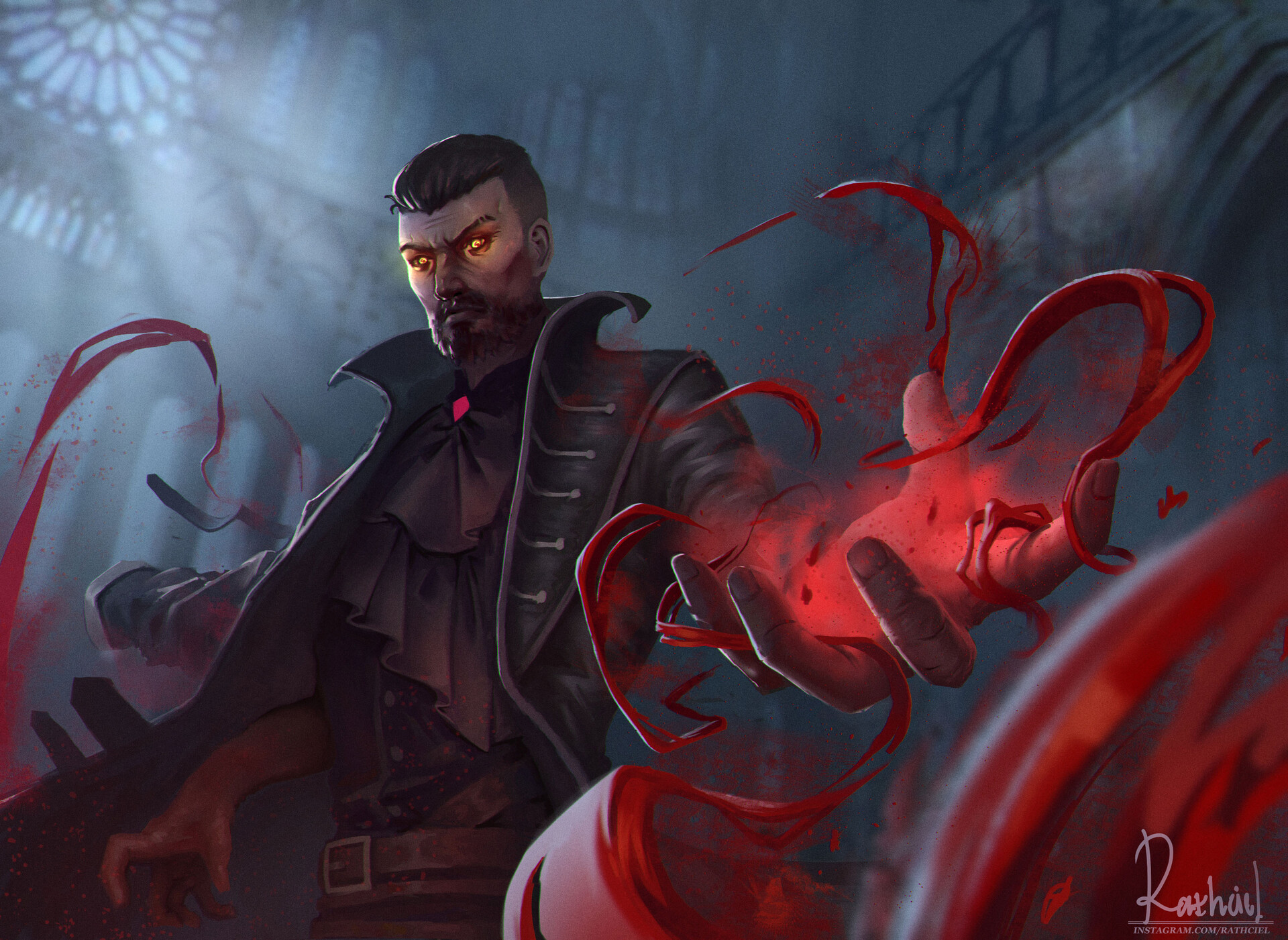This digital artwork depicts a menacing, middle-aged character with a distinct video game/comic book style. The character, who has short, well-groomed dark hair, a beard, and a mustache, stands in a dimly lit castle atrium. He has glowing orange eyes and a scar on his left cheek, adding to his intimidating appearance. He is dressed in a unique 18th-century-inspired outfit, featuring a vampire-like jacket and a black pirate-style shirt. Around his neck, he wears a bright red medallion. His hands are outstretched, emitting a magical red liquid substance that glows in the dark environment. The background showcases a gray, church-like interior with arched windows letting in moonlight. The artwork has a reddish tint throughout and is signed by an artist named Rathail in the lower right corner.